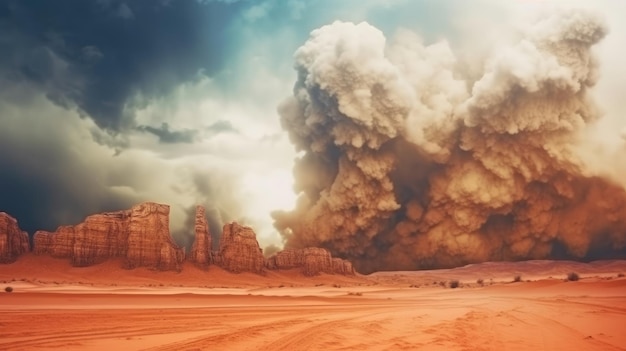The image depicts a dramatic desert landscape with a distinct red sandy foreground that transitions into a vast, flat expanse of reddish sand, almost clay-like in appearance. On the left side of the image, there are rugged canyon rocks, colored with shades of beige and red clay, adding a striking contrast to the arid scenery. The upper left corner of the landscape reveals a dark blue, cloudy sky that progressively deepens to dark gray as you move downward. The right upper portion of the image is dominated by enormous plumes of white smoke, billowing upwards and obscuring the horizon. This cloud of smoke or dust appears immensely large, almost quadrupling the size of the canyon formations, lending a dramatic and dynamic element to the scene. The landscape captures the intense and contrasting elements of a desert environment amidst a dust storm, framed by the tumultuous skies above.